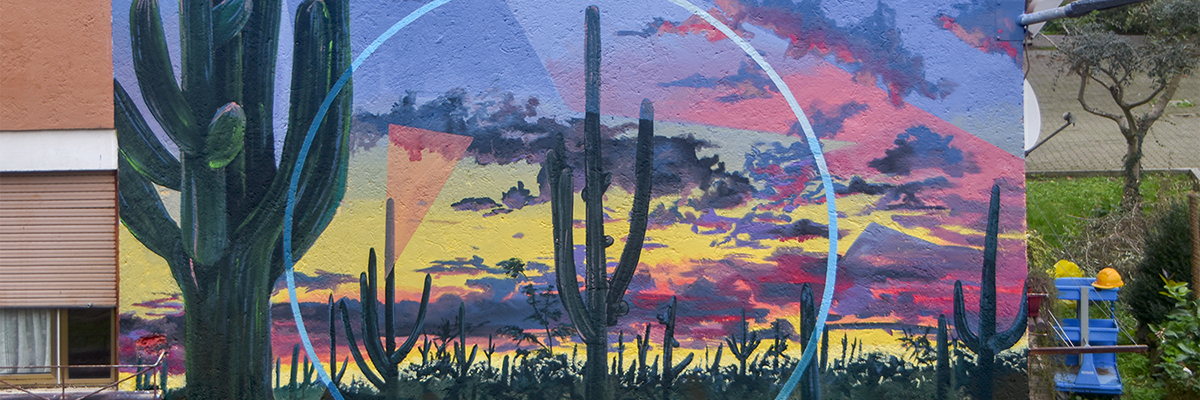The image is a detailed montage blending photographs and a colorized or computerized painting. Central to the image is a large, blue circle, cut off at the top and bottom, that frames numerous tall, dark cacti, likely indicating a desert scene in Arizona. These cacti, rendered in dark black pine green, cast shadows against a vibrant sky transitioning between sunset and sunrise, with shades of yellow, pink, blue, and black clouds. In the background, the cacti diminish in size, stretching towards the horizon.

The left side of the montage displays a mural or painting on the side of a building, featuring a large saguaro cactus in dark forest olive green, accompanied by smaller cacti. The surrounding realistic elements show an outdoor setting with a yard, a tree, a building, a satellite dish, and a blue carrying case. The mural and real-life images combine to create a seamless Southwestern landscape, rich in color and detail, emphasizing the natural beauty of the desert scene.